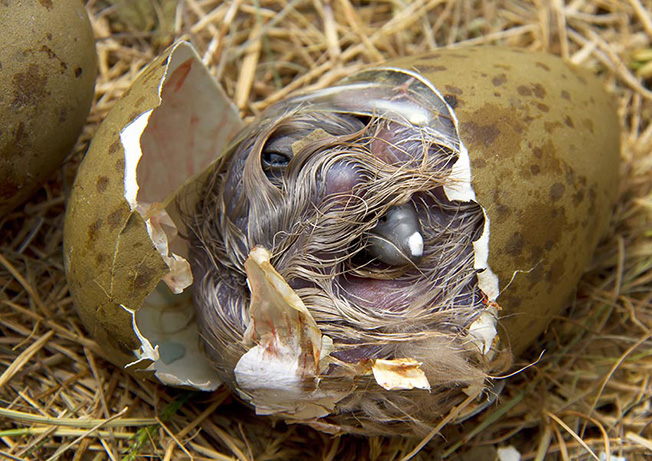The image showcases a medium brown egg with darker brown splotches, nestled on a bed of hay and dried grass. The focus is on the egg, which has cracked open on the left side, revealing a creature amidst the broken shell. The creature inside is mostly a greyish-pink with patches of wet, stringy, hair-like feathers and one visible eye. It appears quite indistinct, though it seems to be a baby bird given the visible beak and the context of the egg. The inner shell is mostly white with some smears of red and blue. Part of another similar egg is visible in the upper left-hand corner, sharing the same brown and splotchy pattern, but its status—whether hatched or intact—is unclear.